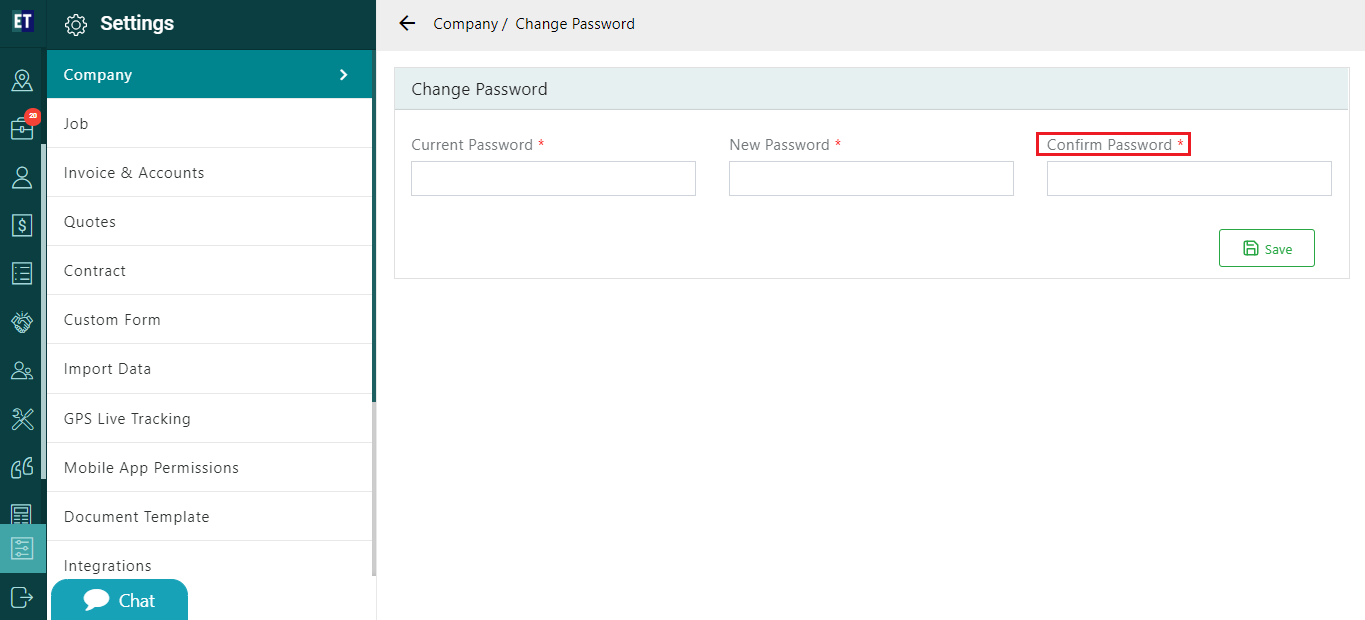This is a screenshot of a web application interface featuring a settings page. The layout is divided into two distinct sections: the left-hand side is adorned with a dark green or turquoise background, while the right-hand side utilizes a palette of primarily gray, light gray, and white tones.

On the left, a vertical toolbar showcases a series of icons symbolizing different functionalities: a person, a map, a briefcase, tools, and quotes. Immediately to the right of this toolbar, the user is navigated to the settings page, prominently indicated by the word "Settings" and a gear icon at the top.

Beneath the heading are the various settings categories listed vertically: Company, Job, Invoice & Accounts, Quotes, Contract, Custom Form, Import Data, GPS Live Tracking, Mobile App Permissions, and Document Template Integrations. Toward the bottom of this list, a blue button offers a chat option for support.

Currently, the "Company" settings category is selected, indicating the user is managing company-related settings. The main section of the page displays options under this category, specifically highlighting the "Change Password" functionality. Three labeled text boxes are aligned horizontally for password management: "Current Password," "New Password," and "Confirm Password," with the "Confirm Password" box outlined in red to possibly indicate an error or required field.